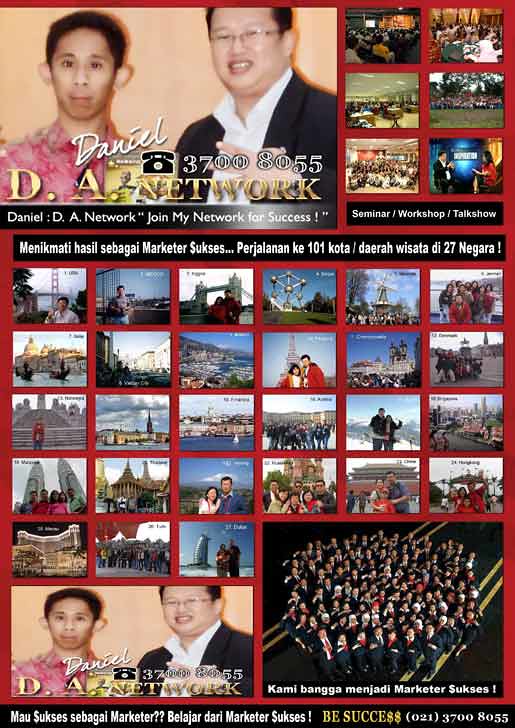The vertically aligned rectangular image is a large, red-backed poster, likely an advertisement or flyer for a seminar or workshop. Prominently featured in the upper left and lower left corners is a rectangular picture of two men, one Asian with glasses and a black suit over a white collared shirt, and the other with darker skin and a red button-down shirt. It reads "Daniel DA Network." The main body of the poster displays organized arrays of smaller images, with two columns of pictures showing various events and people on the right, and rows of images of outdoor locations below, arranged six across in four rows and three in the fifth. The middle of the poster contains white text in a foreign language, which includes phrases like "Menikmati Hasilsebage, marketer suksis, per Jalanen K101 Coda/Dera Wisata D27 Nagara!" Additionally, the English phrases "be success" and a contact number "021-3700-8055" can be seen on the poster. The overall design and content suggest it is an informative piece for a vacation seminar or a similar educational event.